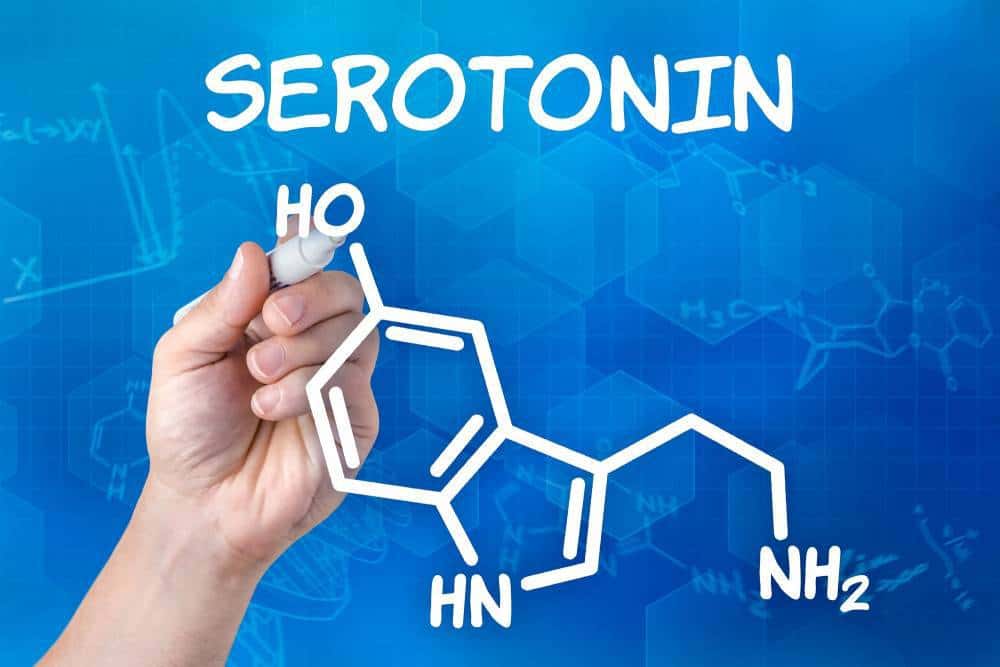The image depicts a digitally created educational slide focused on the molecular structure of serotonin. The background is a blue grid adorned with various scientific calculations, chemistry formulas, and faint graphs. In the top center, the word "Serotonin" is written in white, comic sans-like font. Below, a hand holding a white marker appears to be writing on the screen, illustrating the chemical compound. The molecule is detailed with labels HO at the top, HN to the lower left, and NH2 at the lower right, all aligned in white text alongside the chemical structure. Light blue overlapping diamonds and shades enhance the visual depth, emphasizing the educational and scientific theme of the presentation.